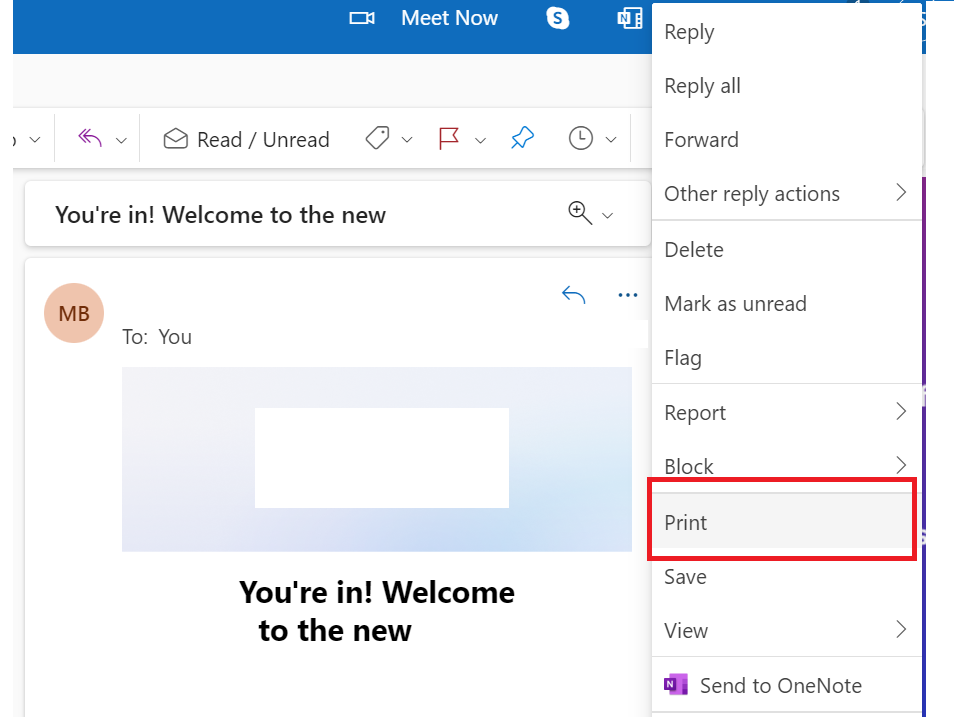This is a detailed screenshot of an Outlook email interface. The image captures a portion of the Outlook email website, showcasing various elements and toolbar options. 

At the top of the screen, there is a small video camera icon accompanied by the text "Meet Now," alongside a Skype icon and a Microsoft OneNote icon. A dropdown menu has been accessed, presenting several options: Reply, Reply All, Forward, Other Reply Actions, Delete, Mark as Unread, Flag, Report, Block, Print, with a red rectangle highlighting the Print option, as well as Save, View, and Send to OneNote.

Additionally, the screenshot reveals part of the email toolbar, featuring buttons like Reply All, Read/Unread, an open email button, as well as icons for tagging, flagging, pinning, and a time clock. 

The email content displayed begins with "You're in, welcome to the new," and to the right, a magnifying glass icon is visible. The sender's icon, labeled "MB," and the recipient information indicate the email is addressed to the user. A blue and white rectangle with "You're in, welcome to the new" in black font is prominently featured. Overall, this screenshot captures a partial view of the Outlook email interface, highlighting both functional and content elements.